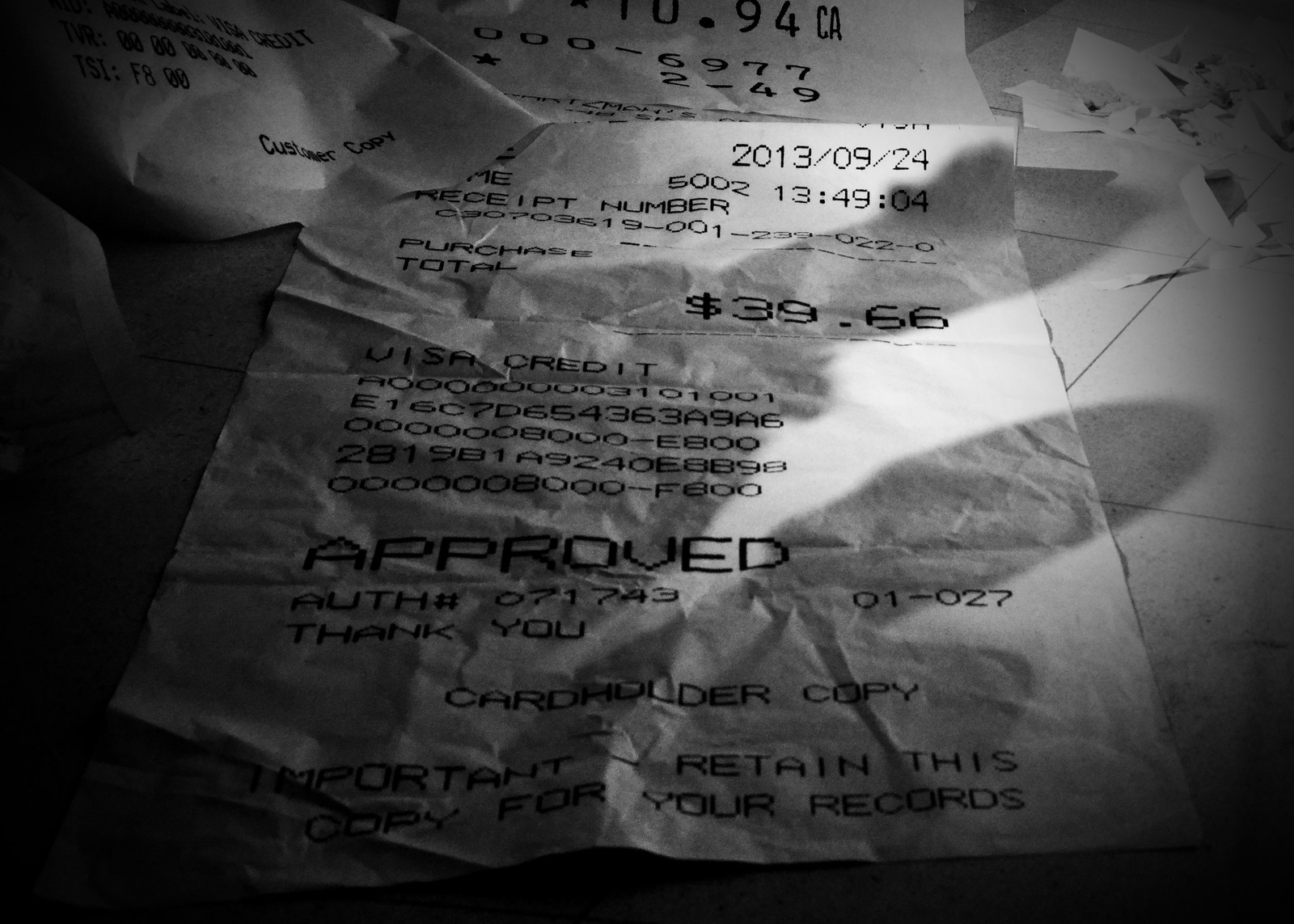The black-and-white image captures a dimly lit scene, featuring a crumpled receipt laid diagonally from the bottom towards the center. This main receipt, dated 2013-09-24, bears a time code of 13:49:04 and a total purchase amount of $39.66. The receipt is a cardholder copy, with "approved" stamped on it in bold letters. The floor beneath is tiled in a white diamond pattern, casting a shadow that obscures parts of the receipt. Additional papers and another less crumpled receipt are visible at the top left and right corners. The image angle is a harsh combination of side and top-down views, accentuating the folds of the receipt, which appears to have been folded several times. Shadows in the lower right corner suggest the presence of people, possibly standing over the scene.